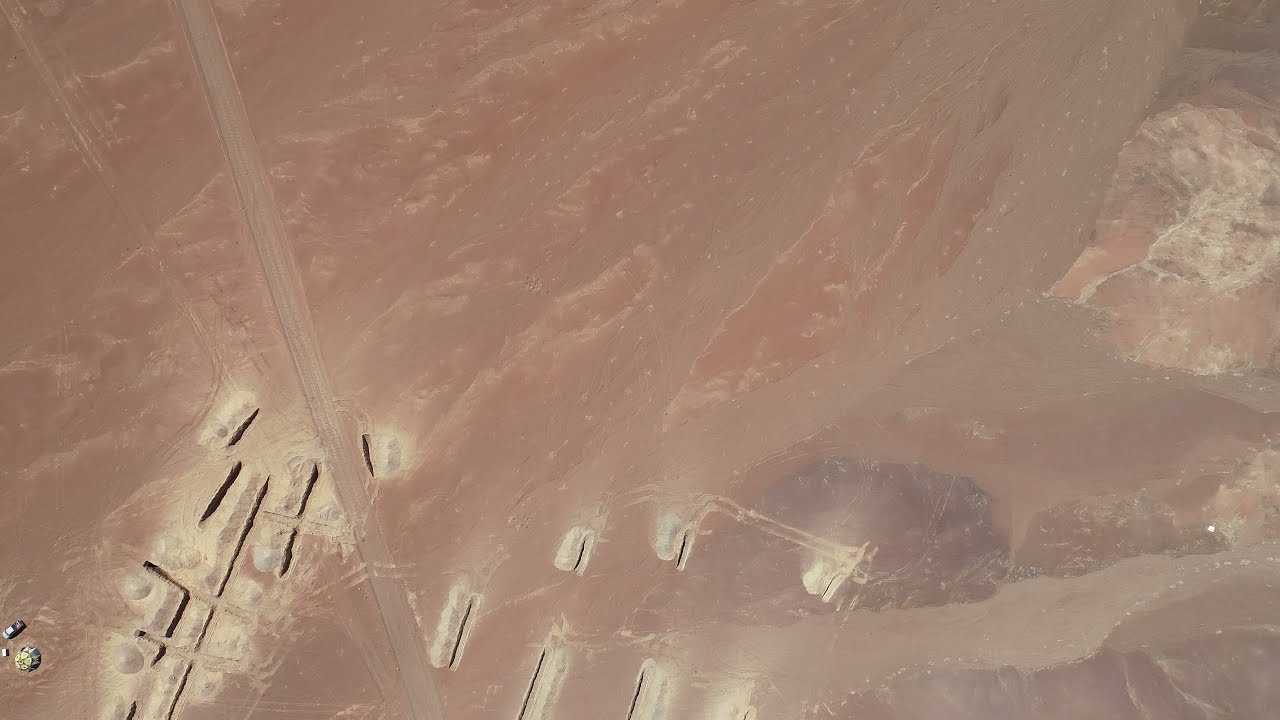The image is an aerial shot, likely taken from a drone or an airplane, capturing a desolate, reddish-brown and gray landscape, characterized by a barren, rocky terrain. The texture appears ambiguous, fluctuating between looking like rock and dirt due to the distance from which the photograph was taken. In the lower left of the image, there are several rectangular carve-outs or divots in the land, suggesting some form of human intervention, possibly building foundations or land parcels. A dirt road cuts diagonally across the scene, running from the bottom left to the top left. This road is complemented by other linear tracks, giving the landscape a segmented appearance. The photograph also reveals a vehicle in the lower left area, positioned near a circular structure, adding to the enigmatic feel of the scene. The overall coloration of the image is a muted maroon with grayish and reddish tones, enhancing its alien, almost Martian-like quality. Small whitish-gray rocks are scattered, particularly noticeable in the upper right portion, providing a contrast to the predominantly monochromatic surface.